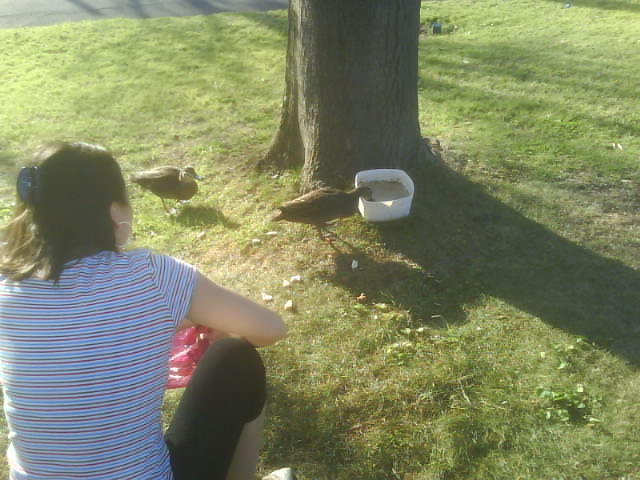In this vibrant park setting, a woman squats on freshly cut, short grass, surrounded by nature. She is wearing black capri pants, white shoes, and a blue and pink striped shirt, with her long brown hair secured by a blue hair clip. In front of her, a large brown tree trunk dominates the center of the image, its base visible and its shadow casting alongside those of the two ducks. A rectangular bucket filled with water sits before the tree, with one brown duck eagerly dunking its head into it, while another duck stands behind, curiously observing. To the top left, a sliver of gray asphalt road is visible, hinting at the park's boundary. The scene captures a quiet, sunny moment of interaction between the woman and the ducks, who seem more interested in the water than any food she might be offering.